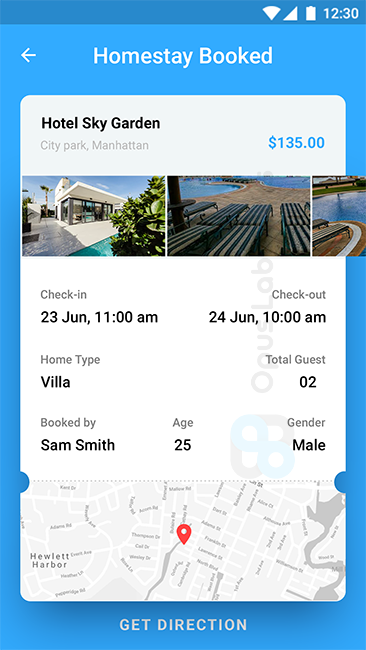This image is a detailed screenshot from a smartphone app, showing information about a booked homestay. The screenshot, captured at 12:30, features a blue background with white text at the top. An arrow icon in the upper left corner enables navigation back to a previous screen, while the central heading reads "Homestay Booked."

Prominently displayed is a sizable white rectangle containing key booking details: 
- Hotel Sky Garden, City Park, Manhattan
- Price: $135

Beneath this, the screenshot includes three photographs:
1. An outdoor view of a pool house adjacent to a swimming pool.
2. A set of outdoor lounge chairs situated on what appears to be a beach.
3. A poolside perspective featuring the same lounge chairs.

Additional booking information follows:
- Check-in: 23 June, 11 a.m.
- Check-out: 24 June, 10 a.m.
- Home Type: Villa
- Total Guests: 2
- Booked by: Sam Smith, Age: 25, Gender: Male

Further down, there's a road map, likely from Google Maps, highlighting the location with a red icon.

Returning to the blue background, the scene concludes with white text prompting "Get Direction."